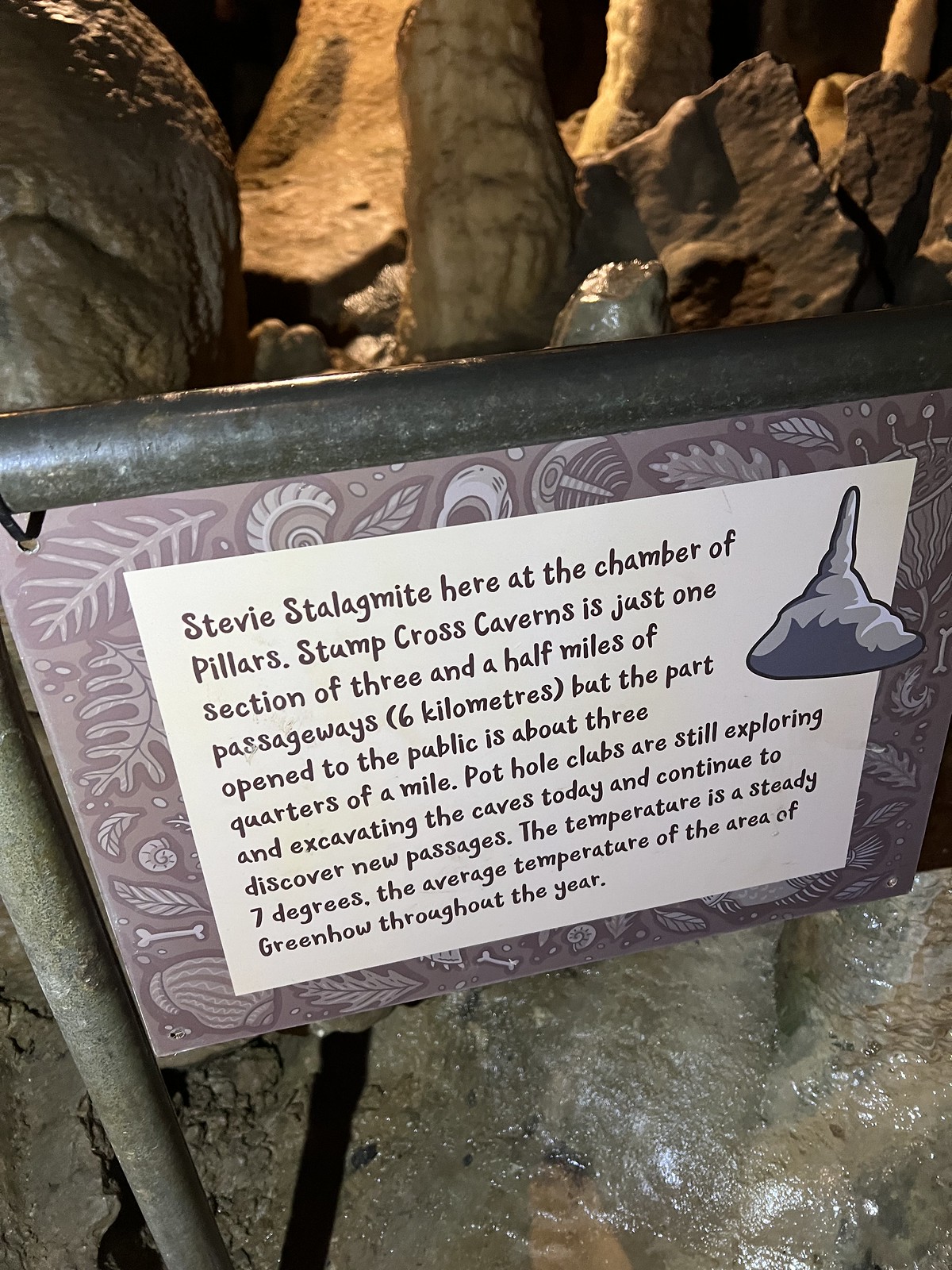The image is a color photograph in portrait orientation, depicting an informational sign within a stalagmite cave. The setting is a wet, rocky area inside the cave, with various stalagmite formations visible in the background. The ground surface appears moist, and the air is likely cool with a steady temperature of seven degrees Celsius, typical of greenhouse conditions throughout the year.

Prominently positioned in the center of the image, the sign is mounted on a rusty dark gray metal pole. The sign itself features a mauve border adorned with illustrations of leaves and shells, suggesting possible petrification. Within this border, a white rectangle holds black lettering and a line art illustration of a stalagmite in the top right corner. The text reads: "Stevie Stalagmite here at the Chamber of Pillars. Stump Cross Caverns is just one section of three and a half miles (six kilometers) of passageways, but the part open to the public spans about three-quarters of a mile." Additional sentences on the sign mention ongoing exploration and excavation by pothole clubs, which continue to unveil new passages within the cave system. The photograph captures the realism of the setting, highlighting the natural and man-made details within this subterranean environment.